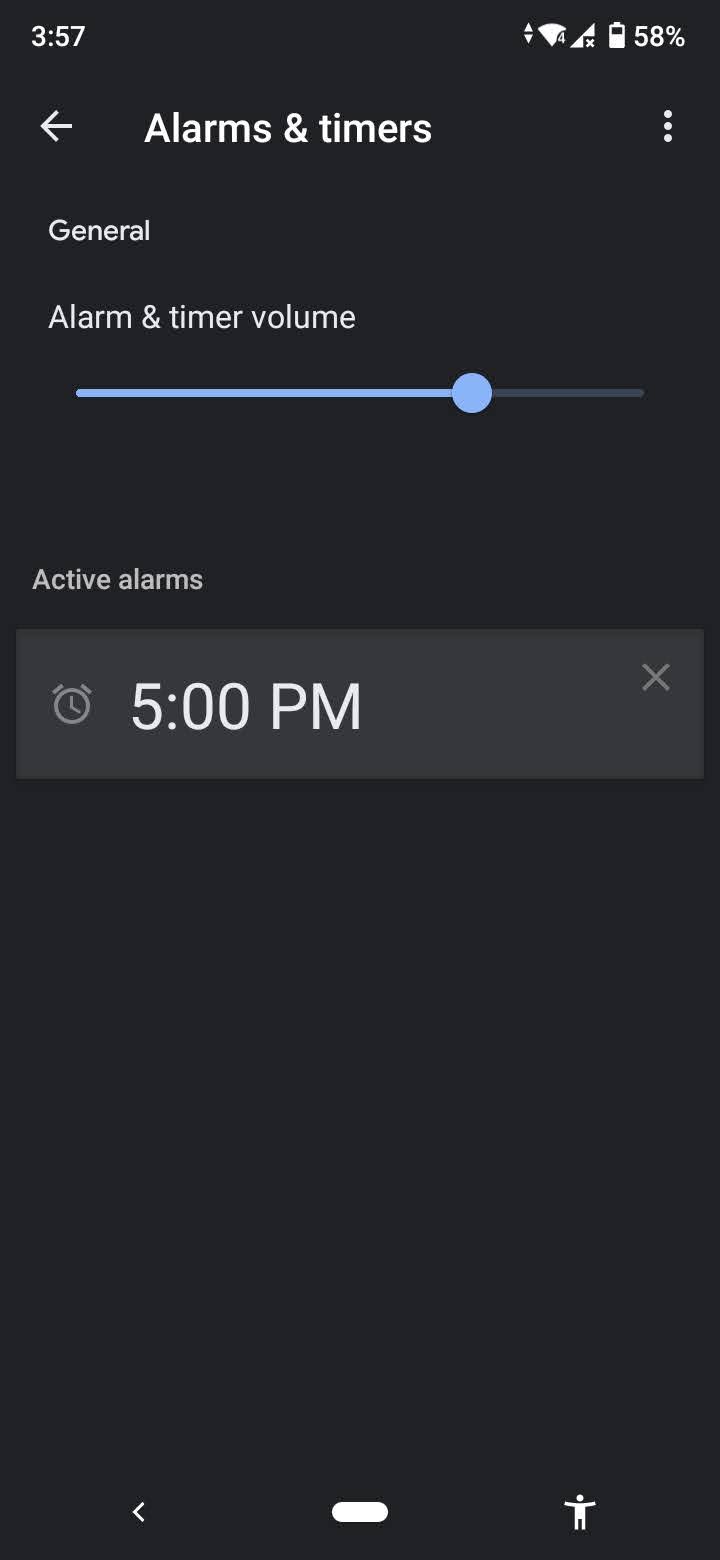This is a highly detailed screenshot of a clock application on a mobile phone with a dark grey background. The top section features standard phone icons, with a white, left-pointing arrow on the left side, and to its right, the text "Alarms and Timers" in white. Following a gap, three vertically stacked white dots appear on the right.

Below, small white text reads "General" on the left, followed by "Alarm and Timer Volume" underneath. A slider bar is situated below, colored light blue on the left, transitioning to dark grey on the right, marked by a light blue circle indicating the current volume level.

Further down, the label "Active Alarms" appears in white on the left. Directly beneath this, there is a dark grey rectangular box. On the left side of this box, a light grey alarm clock icon is visible. To the right of the icon, white numerals and text display "5 PM." In the top right corner of the same box, a light grey 'X' is located. 

Considerable negative space with a dark grey background follows this section. At the bottom of the screen, three icons are presented: a left-pointing white arrow, a white pill shape in the center, and a white icon resembling a person with outstretched arms on the right.

At the very top left, the time is shown as "3:57." The top right corner, from right to left, indicates "58%" next to a vertical battery icon about 58% filled with a white bar, along with a couple of additional icons.